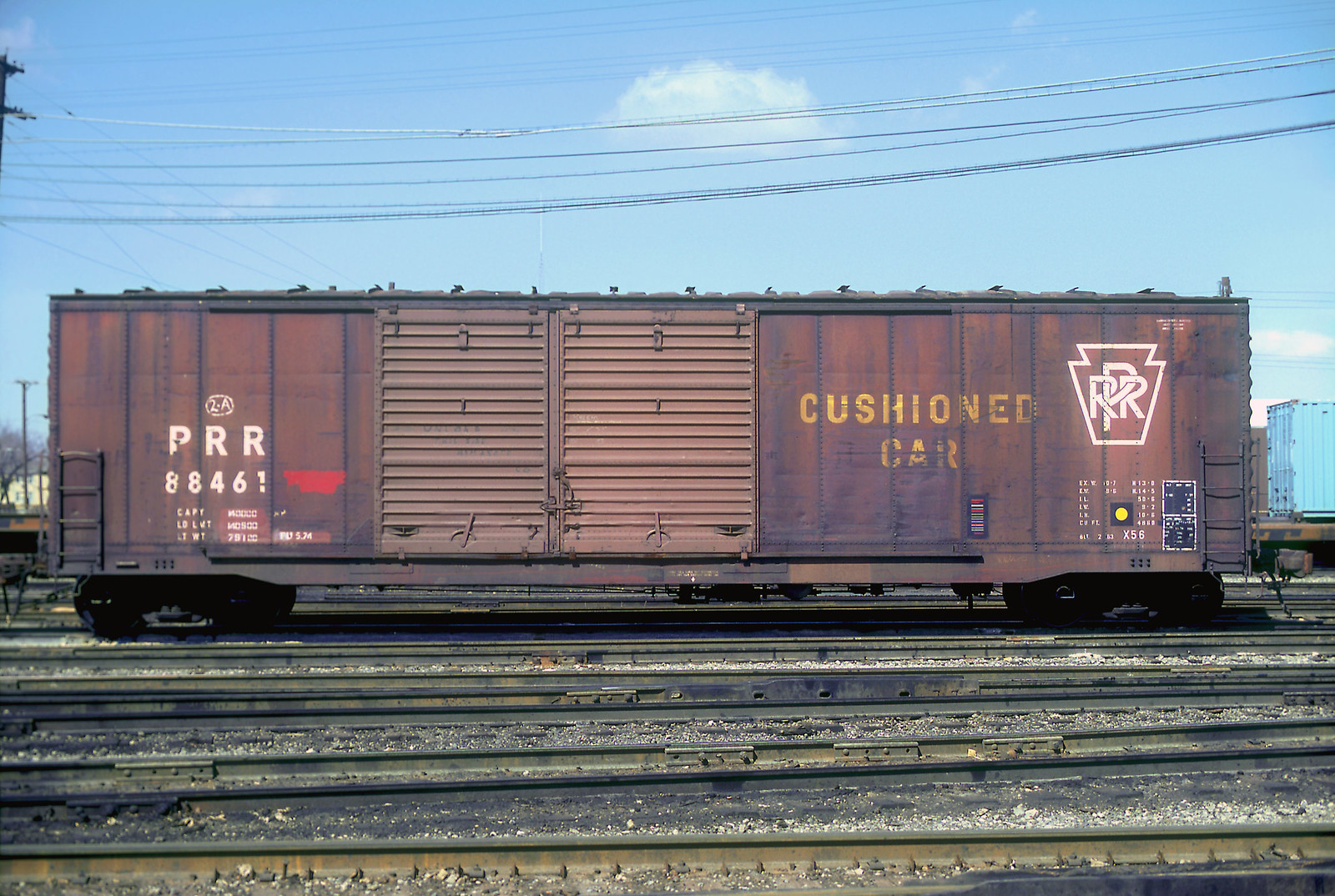The photograph captures a single, rust-colored train car, designated with the white lettering "PRR 88461" on the left and "Cushion Car" in yellow letters towards the center right. The car also features a white PRR logo with a pyramid-like outline to the far right. The train car is positioned on multiple steel tracks that span horizontally across the foreground. In the background, a partly cloudy blue sky and several power lines stretching from left to right frame the scene, along with a utility pole partially cropped on the left. The ground is covered in gravel and dirt, and there is a glimpse of a light yellow train car mostly cropped out to the far right. The image is naturally lit, suggesting it was taken during the daytime.